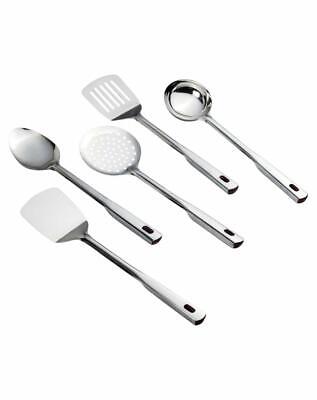This is a polished stainless steel set of five large cooking utensils laid out diagonally from the lower right to the upper left on an all-white background, giving it a clean product photo look. The utensils, arranged in a slightly staggered line with even-numbered utensils slightly higher than the odd-numbered ones, feature long, narrow rectangular handles with holes for hanging. From bottom to top, the set includes: a fully covered flat spatula for flipping eggs, a large solid spoon for stirring soups, a round strainer resembling a flat coaster with holes for draining, a slotted spatula ideal for flipping greasy foods, and at the top, a ladle for scooping liquids. The highly reflective, bright shine of the stainless steel highlights the quality and sophistication of these essential kitchen tools.